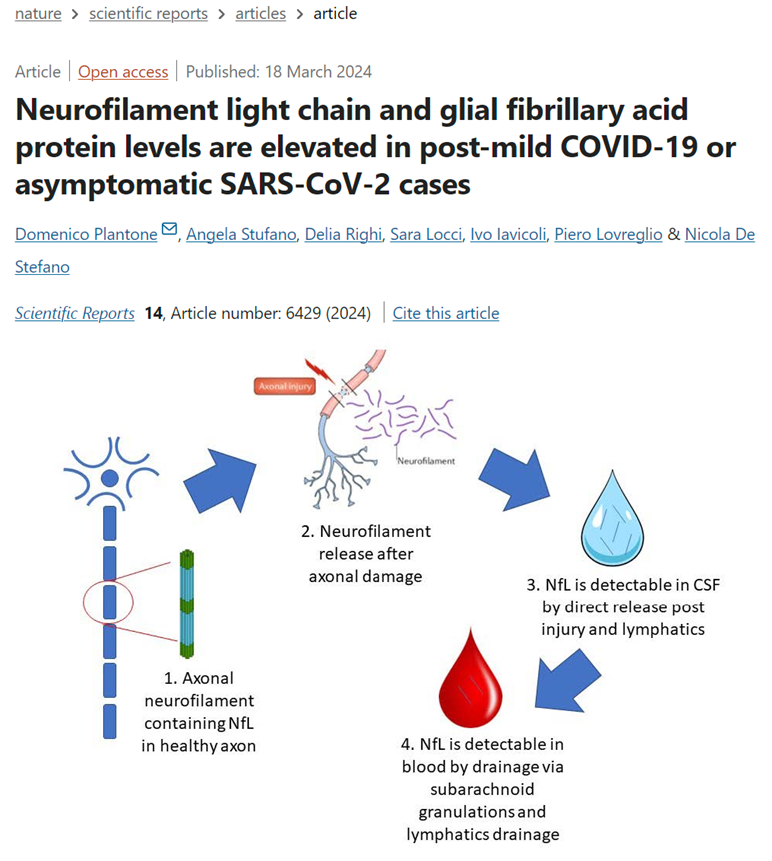This image is a screen capture of a scientific article published on March 18, 2024, in "Nature, Scientific Reports." The article, titled "Neurofilament Light Chain and Glial Fibrillary Acid Protein Levels Are Elevated in Post-Mild COVID-19 or Asymptomatic SARS-CoV-2 Cases," is authored by Domenico Plantone, Angela Stufano, Delia Ruhi, Sarah Loshi, Eva Chioli, Piero Lovreggio, and Nicola De Stefano. The citation is "Scientific Reports 14, Article Number 6429, 2024."

The image includes a diagram with a white background illustrating the progression and detection of neurofilament light chain (NFL) after axonal damage, specifically in relation to COVID-19. There are four key steps shown with corresponding blue arrows. 

1. An initial depiction of a healthy axon labeled "Axonal neurofilament containing NFL," visualized with blue dots forming a vertical line and both green and blue elements.
2. Neurofilament release after axonal damage, represented by red and blue structures that resemble veins or stems.
3. NFL detectable in cerebrospinal fluid (CSF) by direct release post-injury via lymphatics, depicted as a large blue teardrop with an arrow pointing to it.
4. NFL detectable in blood by drainage via subarachnoid granulations and lymphatic drainage, shown as a red teardrop with the final blue arrow indicating this step.

The diagram visually summarizes the process from healthy neurofilaments contained within axons to their detectable presence in CSF and blood following axonal injury.